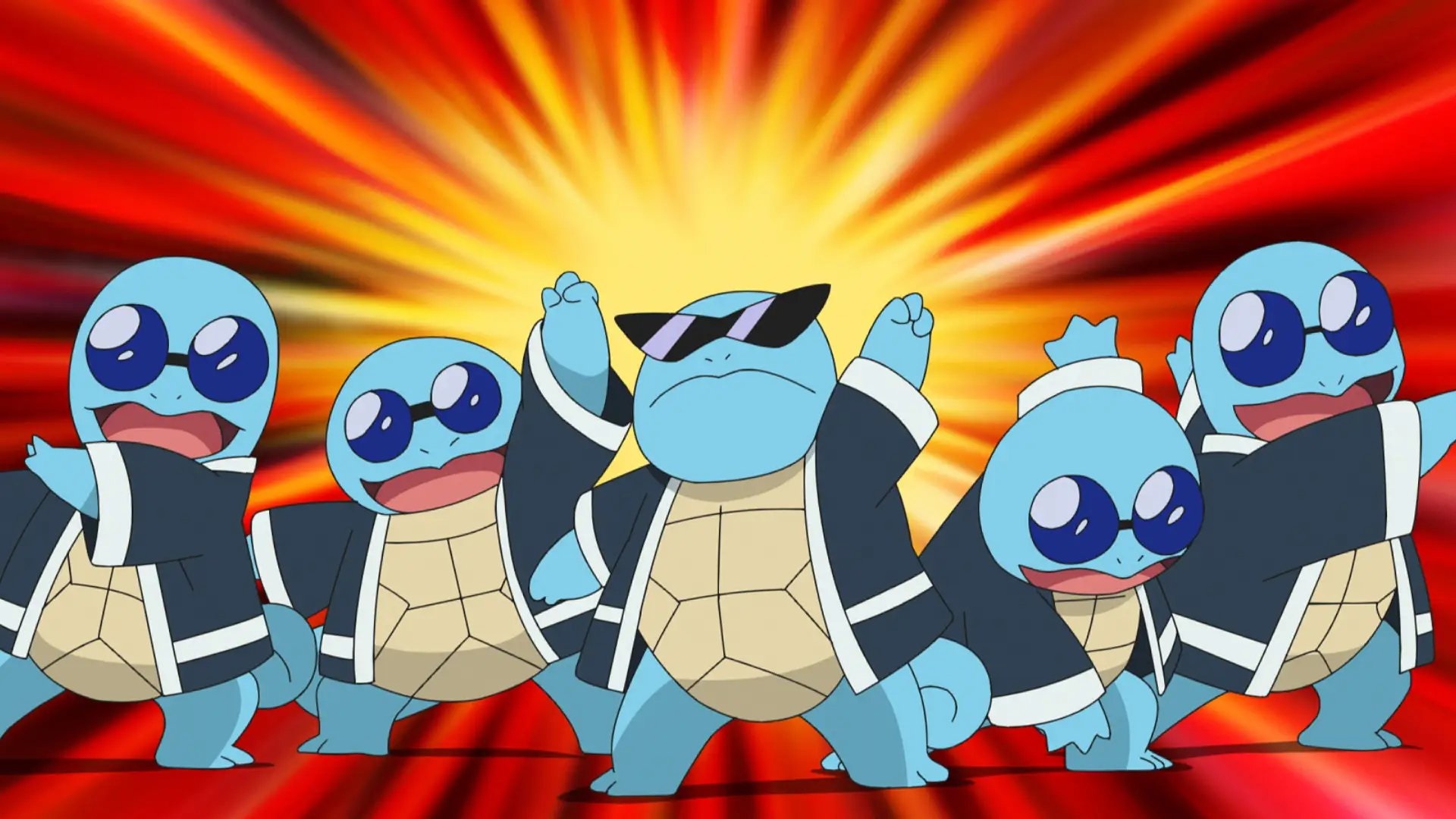This vibrant screenshot from the cartoon Pokémon captures a dynamic scene featuring five Squirtles, turtle-like creatures known for their watery abilities. In a formation reminiscent of a performing band, the Squirtles are striking various energetic poses against a radiant backdrop. The background displays a dramatic sunburst effect with yellow at the center, radiating outward with orange and red lines, enhancing their dynamic appearance.

All five Squirtles are clad in coordinated dark blue happi coats with white trims on the hems, pockets, and sleeves. The four Squirtles on the sides don matching round blue sunglasses, while the central Squirtle stands out with striking black, triangular sunglasses. This Squirtle, positioned at the forefront, is distinguished not only by its unique eyewear but also by its confident stance, with one hand pointing upwards and the other downwards, exuding a sense of leadership and camaraderie among them. The scene has a nostalgic, showbiz feel, evoking the image of a classic performance group ready to take the stage.